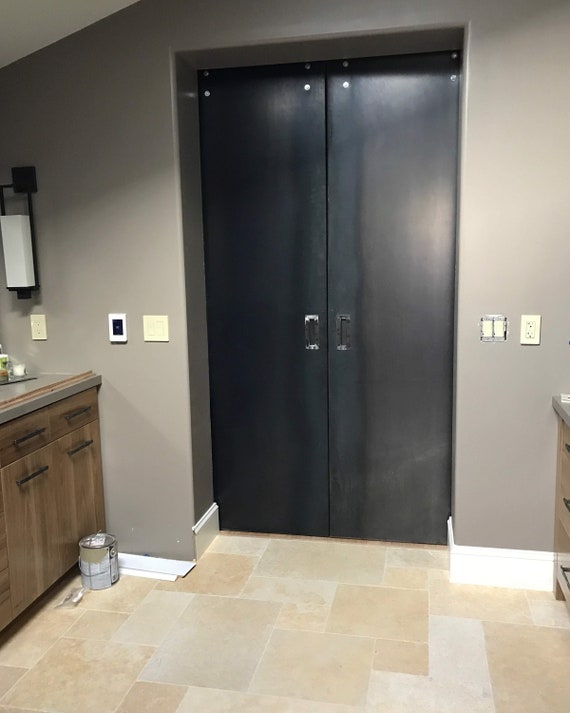This is a full-color photograph taken indoors using artificial light. The vertically rectangular image captures what appears to be a bathroom or kitchenette area with notable beige and gray elements. The room features a dark black double-sided French door with pull handles, positioned centrally within the beige-tan, slightly gray walls. Light switches flank both sides of the door, and electrical outlets are also visible.

The tiled floor comprises a mix of white and brown tiles, bordered with white baseboards. To the left and right of the doors are countertops, with the right side also displaying drawers, cabinets, and a can of paint, which has dripped onto the floor. The photograph might also capture a partial view of a sink near the right-side countertop. The scene is detailed with remarkable contrast provided by the solid tall black doors against the room's predominantly beige tones.